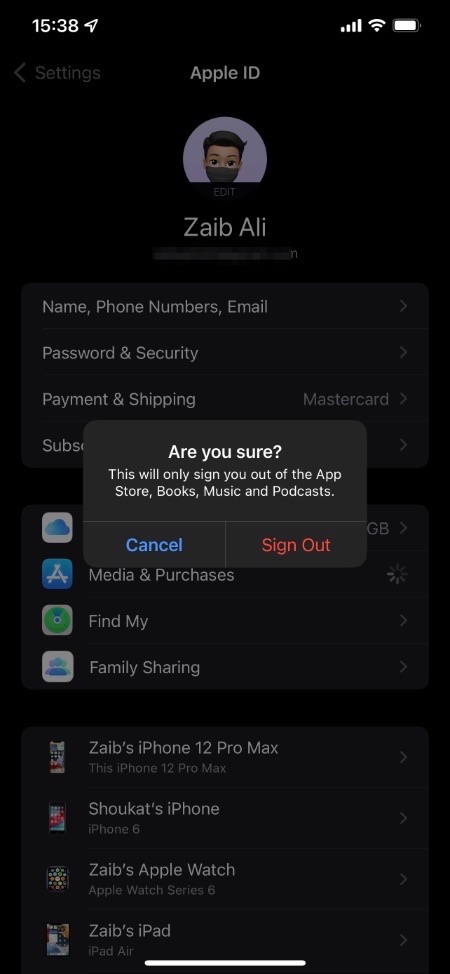This image is a screenshot taken from a smartphone in night mode, which gives the background a deep black hue. Displayed at the top of the screen is the device's clock showing the time as 15:38. The screen captures the Apple ID settings window, signifying that the user has several Apple devices and services linked to their account. 

At the forefront, there is a prominent pop-up window asking for confirmation with the message: "Are you sure? This will only sign you out of the App Store, Books, Music, and Podcasts." The window offers two options: "Cancel" in blue text and "Sign Out" in red text.

In the top section of the screen's main content, there's an Apple ID logo featuring an emoticon character in a half-circle with a blue background, wearing a mask. The associated name is "Zabali."

Visible behind the pop-up are various Apple ID settings categories, including:
- Name, Phone Numbers, Email
- Password & Security
- Payment & Shipping
- Media & Purchases
- Find My
- Family Sharing

Additionally, it shows a list of devices associated with the account:
- Zab's iPhone 12 Pro Max
- Shukat's iPhone
- Zab's Apple Watch
- Zab's iPad